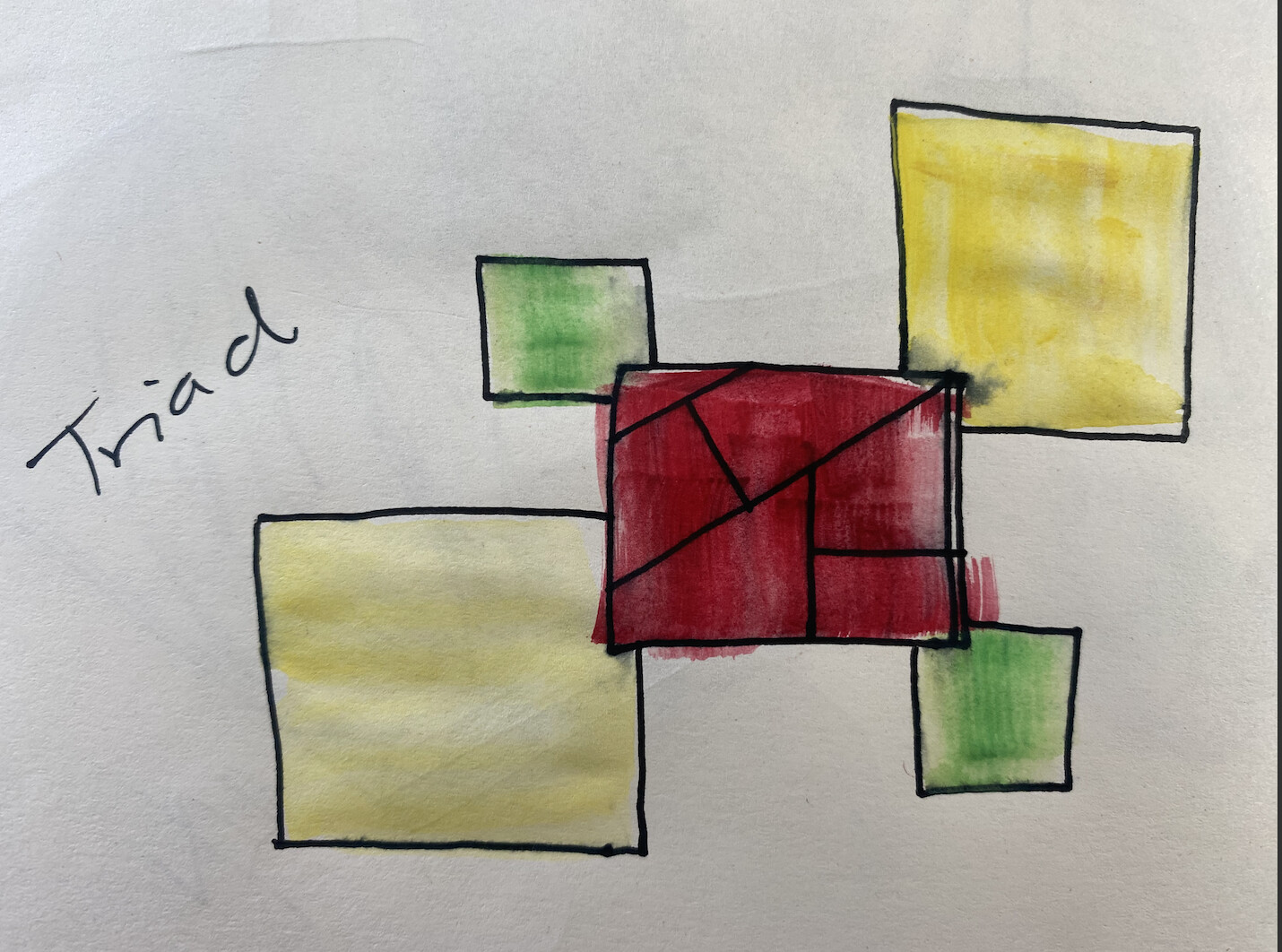This image showcases a sheet of white paper that exhibits visible folds near the middle and top, giving it a slightly worn appearance. Through the paper, you can faintly discern some translucent drawings on the reverse side. 

Dominating the central area of the sheet are five squares, each carefully drawn with black marker. These squares feature distinct colors: two are green and two are yellow. The green squares are positioned diagonally opposite each other. The yellow squares are also placed diagonally but in a slightly different arrangement – one is located at the top left corner and the other at the bottom right corner. Notably, the bottom right yellow square is larger than the top left one.

Centrally located among these squares is a prominent red square. This vivid square is detailed with several black lines that subdivide it into various geometric shapes, including rectangles and trapezoids, as well as partial trapezoids. The colored areas of the squares are meticulously filled using corresponding markers, enhancing the vividness of the design.

On the right side of the paper, the word "triad" is prominently written, blending red and black colors to striking effect. The arrangement and color scheme of the squares, coupled with the word "triad," suggest a thoughtful and deliberate artistic composition.